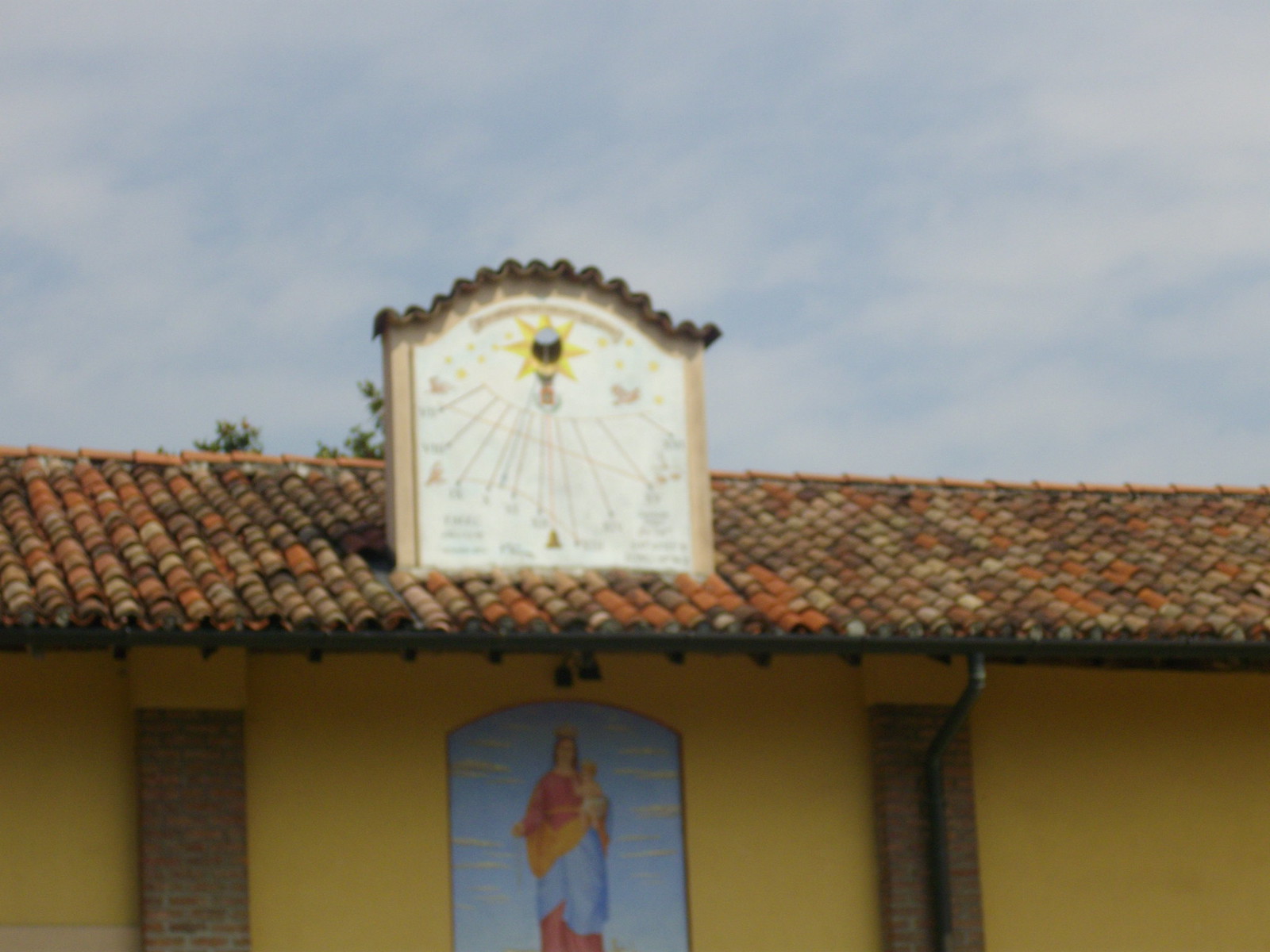The photograph depicts the side of a building, likely a Catholic church or mission, featuring a distinctive, multicolored clay-tiled roof. The roof tiles range in color from brick red to various shades of brown, forming a pattern with oval shapes. The sky above is blue with wispy white clouds, indicating clear weather.

The building itself is painted a medium yellow and includes two brick pillars flanking a central, religious mural. This mural, set against a blue background with cloud-like designs, portrays the Virgin Mary holding baby Jesus. Mary is adorned in a long, flowing robe of white, yellow, and blue, and she wears a crown. Above the painting, the slanted roof features a square ornament with a curved top, embellished with intricate, colorful designs.